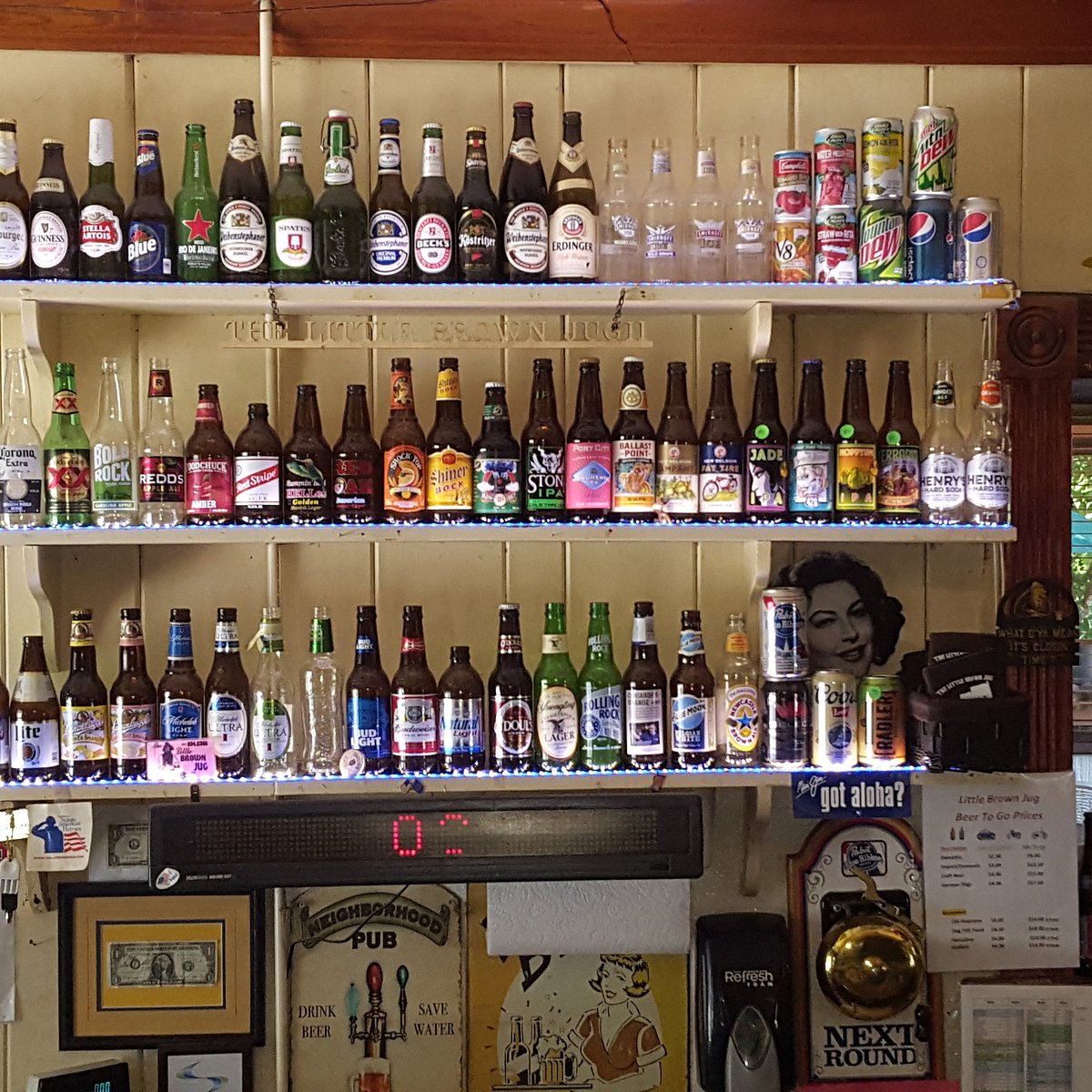In the photo, a set of three white plank shelves are mounted on the wall behind a bar. Each shelf is densely populated with an array of bottles and cans, some empty, some still sealed. The top shelf features a mixture of brands, including clear bottles, brown and green beer bottles, and recognizable soft drink cans such as Diet Mountain Dew, Diet Pepsi, regular Pepsi, and regular Mountain Dew. It also sports a metal sign reading "The Little Brown Jug, 11." 

The middle shelf holds mostly empty alcoholic beverage bottles—brown, green, and clear—including various types of beers like IPA and hard soda. The bottom shelf similarly displays different brands of beer bottles and a few beer cans. A black digital sign with red dot lettering hangs beneath this shelf, displaying a partially visible number. 

In addition, the decor includes a framed $1 bill and a quirky sign that reads, "Neighborhood Pub, Drink Beer, Save Water." There's also an old-fashioned screen for ticket numbers, a hand sanitizing dispenser, and a sign with a bell labeled "Next Round." Hanging on the wall behind the shelves is a black and white photo of a woman's face reminiscent of Ava Gardner, peeking out, and a 40s or 50s comic-style picture of a lady with a tray of beer bottles and a stein. On the far right side, a printed sign details "Little Brown Jug, Beer To Go Prices."